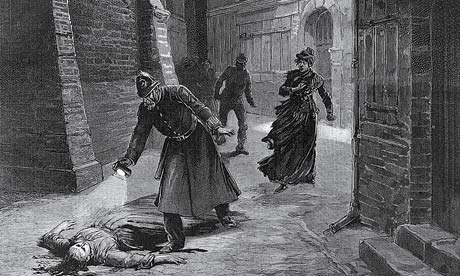This detailed black-and-white sketch captures a haunting scene reminiscent of old London during the Jack the Ripper era. A Scotland Yard policeman, identifiable by his traditional long dress coat and cap, is bent over, intently shining a flashlight on the lifeless body of a woman lying in a narrow, twisting alleyway. The officer’s flashlight creates stark shadows, highlighting the grim nature of the scene. To their left, the aged buildings typical of London’s backstreets rise ominously. In the background, a woman in a black dress clutches her chest, her eyes wide with horror, while further back, a masked man rushes toward the scene. The overall atmosphere is one of tension and dread, evoking the fear and mystery of the Jack the Ripper period.